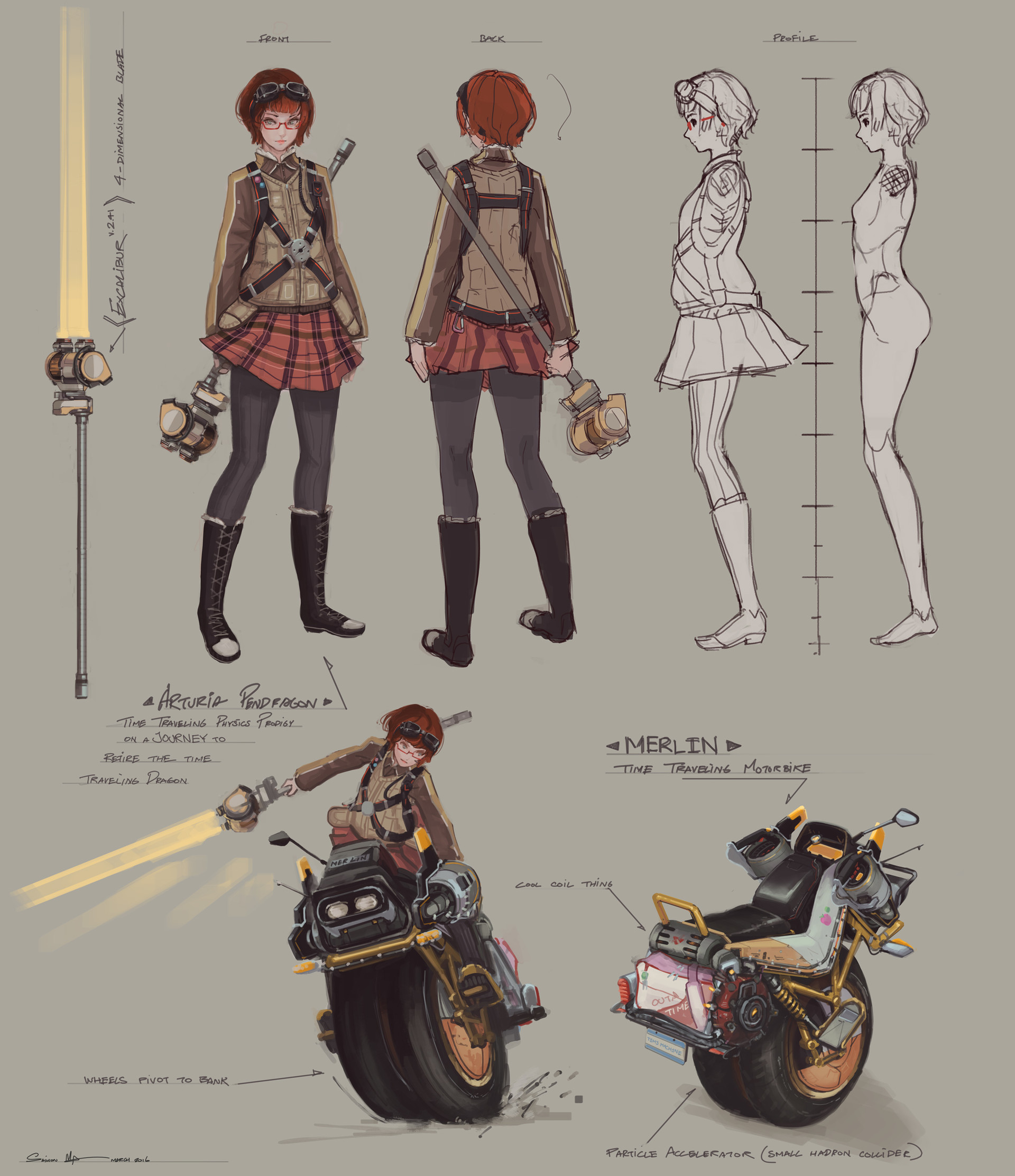The concept art depicts a character named Arturia Pendergon in detailed illustrations from various angles. Arturia sports a brown leather jacket with crisscrossed straps, a red or light brown miniskirt with black stripes, and black long boots over grey tights. She has brown short hair and wears black goggles on her forehead. Her weapon, which appears to be a hammer that transforms into a four-dimensional blade with a spotlight at the end, is strapped to her back. The top row of images presents Arturia from the front, back, and side views, with the side view rendered in black and white. The bottom section showcases Arturia riding a unique one-wheeled motorcycle called Merlin. The artwork also includes measurements and outlines, mapping out her overall design and dimensions.